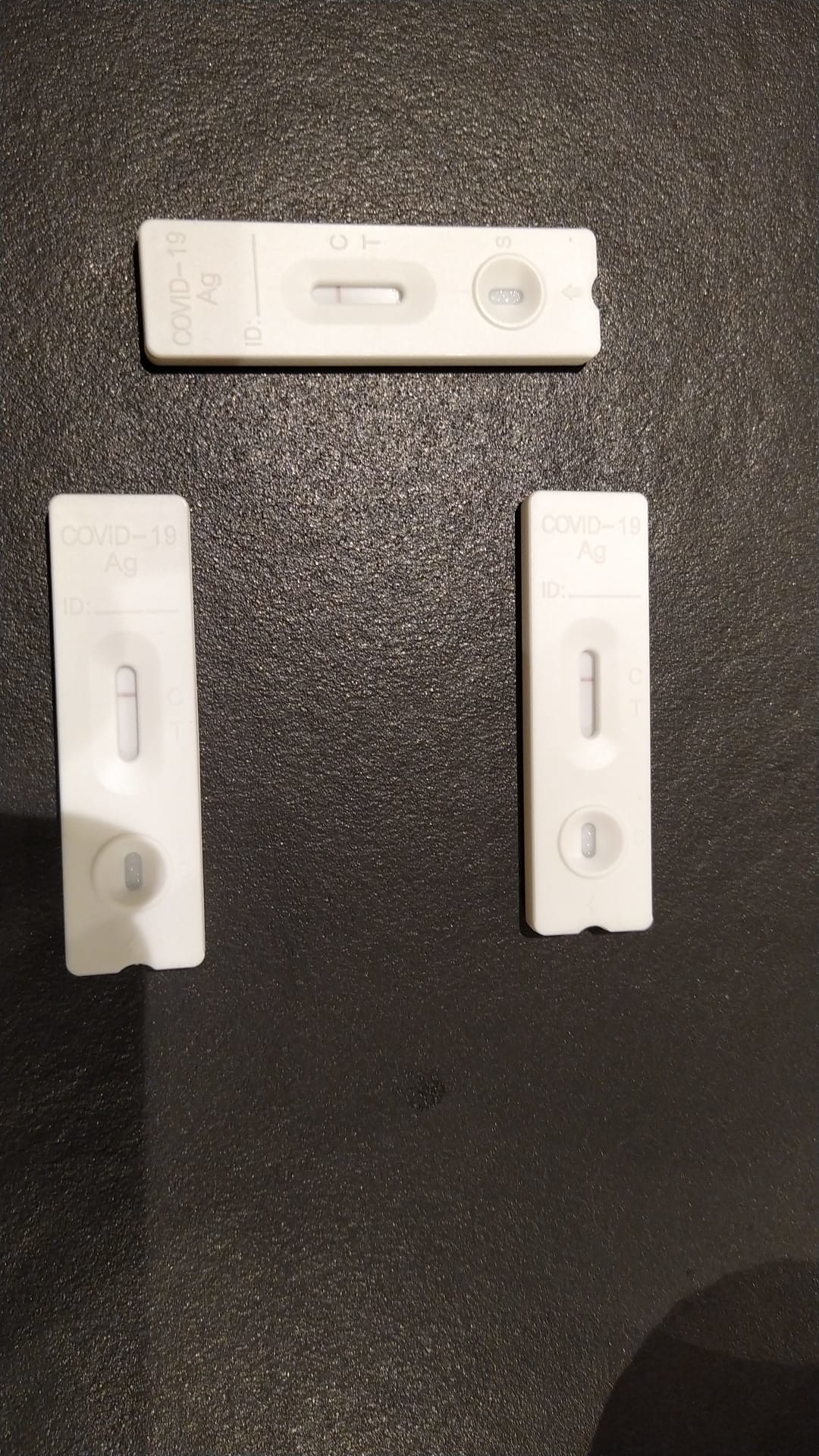The image features a black textured background showcasing three white plastic COVID-19 tests. The tests are labeled at the top with "COVID-19" and beneath that "Ag." Each test includes a section labeled "ID:" followed by a line for writing.

- The first test is long and narrow, positioned horizontally at the top of the image.
- The remaining two tests are in the center, positioned vertically. These tests are wider and shorter but still rectangular.

All three tests have a central, elongated oval section with a pink line near the top. On the right side of this section, the letters "C" (above) and "T" (below) are visible. Beneath the oval section, there is a smaller, rounded square area marked with an "S" on the right side.